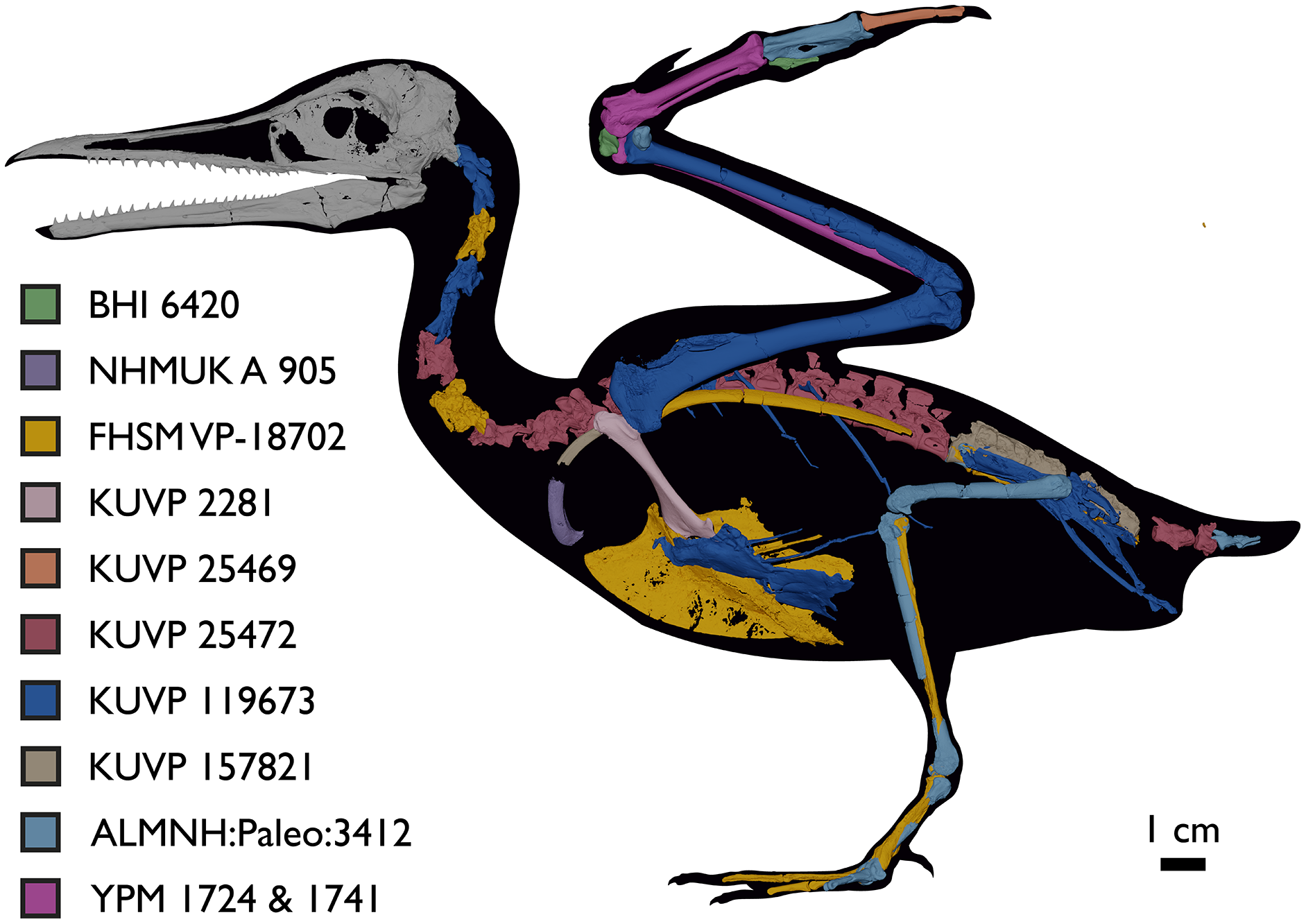This is a detailed cutaway anatomical illustration of an ancient, non-modern bird featuring a black silhouette with a highly detailed color-coded skeletal structure visible inside. The bird, which has a distinctive, elongated sawtooth beak and resembles a hybrid between a turkey and a vulture in body style, is facing to the left. The bird's bones are shown in various vibrant colors, including green, purple, yellow, brownish-orange, dark pink, and multiple shades of blue, purple, and tan. These colors correspond to a comprehensive key located on the left side of the image, with each color linked to specific letter and number combinations (e.g., BHI 6420, NHMUKA 905, FHSMVP 18702). The image incorporates a 1-centimeter scale in the lower right corner, suggesting fine scale measurements. The diagram is laid out in landscape mode against a black background, which accentuates the multicolored bones. This visually engaging schematic, reminiscent of an x-ray, is the type of educational tool you'd find in a textbook, designed to help learners understand the intricate details of avian skeletal anatomy.